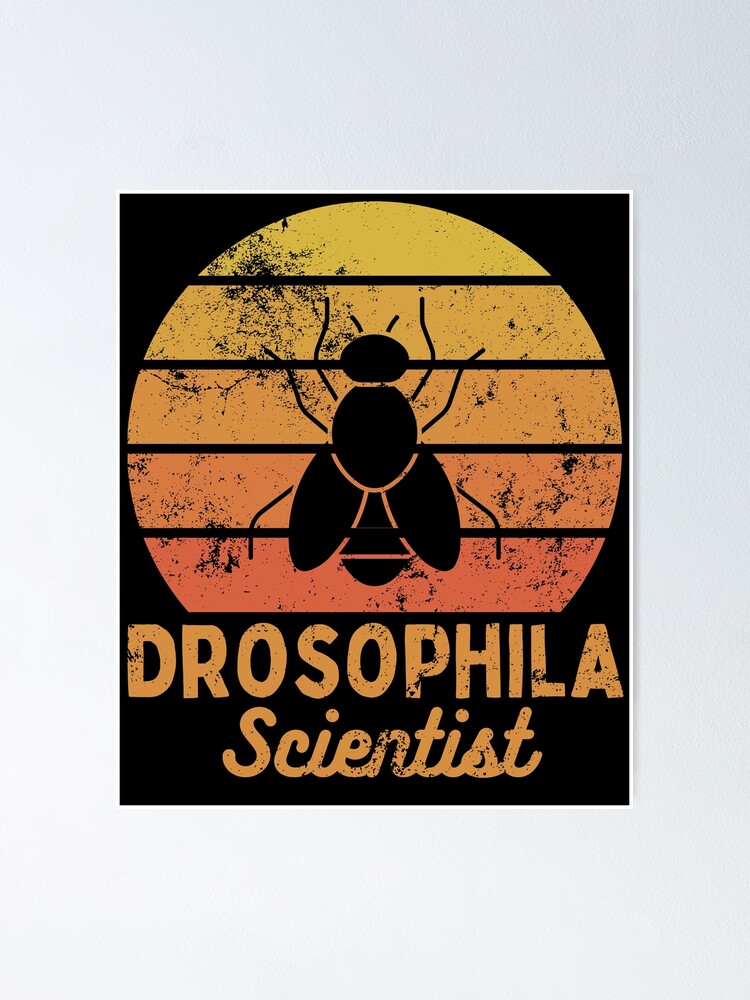The rectangular graphic, taller than it is wide, features a minimalist design with a light gray background. Centered on this gray canvas is a smaller black rectangle, bordered by a thin white line. Inside this black frame, bold orange letters spell out "DROSOPHILA" in block style font at the bottom, with "scientist" elegantly written in cursive beneath it. Above the text, a circular motif occupies the upper portion, segmented into five gradient sections that transition from bright yellow at the top through shades of orange to a deep pink at the bottom. At the center of the circle, a detailed black outline of a fly, complete with six legs, two antennae, a round head, body, and two wings, is prominently displayed. This striking arrangement of text and imagery resembles an emblem or logo, possibly suitable for a scientific advertisement or magazine feature.